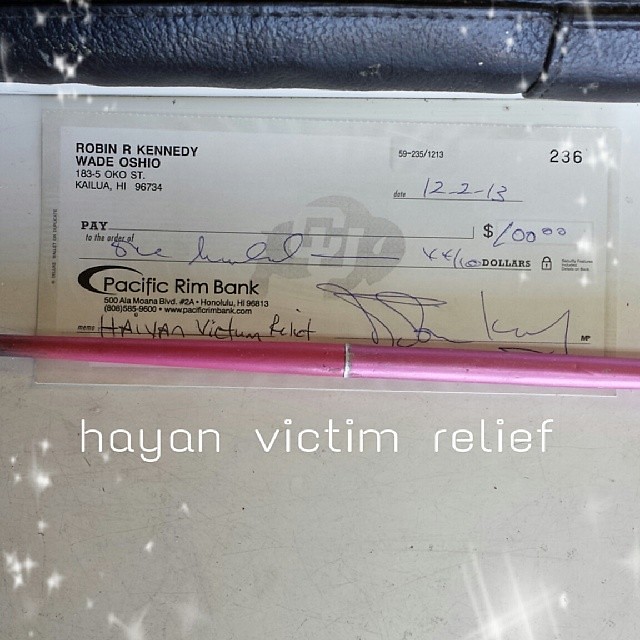The image is a large, square, close-up photo of a personal check lying on a light gray table, partially enclosed by the edge of a black leather wallet with visible stitching at the top. The check is issued by Pacific Rim Bank, located at 500 Ala Moana Boulevard, No. 2A, Honolulu, Hawaii 95813, with contact details 808-585-9500 and www.pacificrimbank.com. The check, numbered 236, is dated December 2, 2013, and made out for $100, although the pay-to-the-order-of line is left blank. The memo line indicates "Hayen Victim Relief." The top left corner of the check lists the names Robin R. Kennedy and Wade Oshio along with the address 1835 Oko Street, Kailua, Hawaii 96734. A pink pen lies across the bottom, obscuring the account and routing numbers. The background of the check subtly features the University of Colorado Buffaloes logo. Overlaid in white lettering at the bottom of the image is "Hayen Victim Relief."